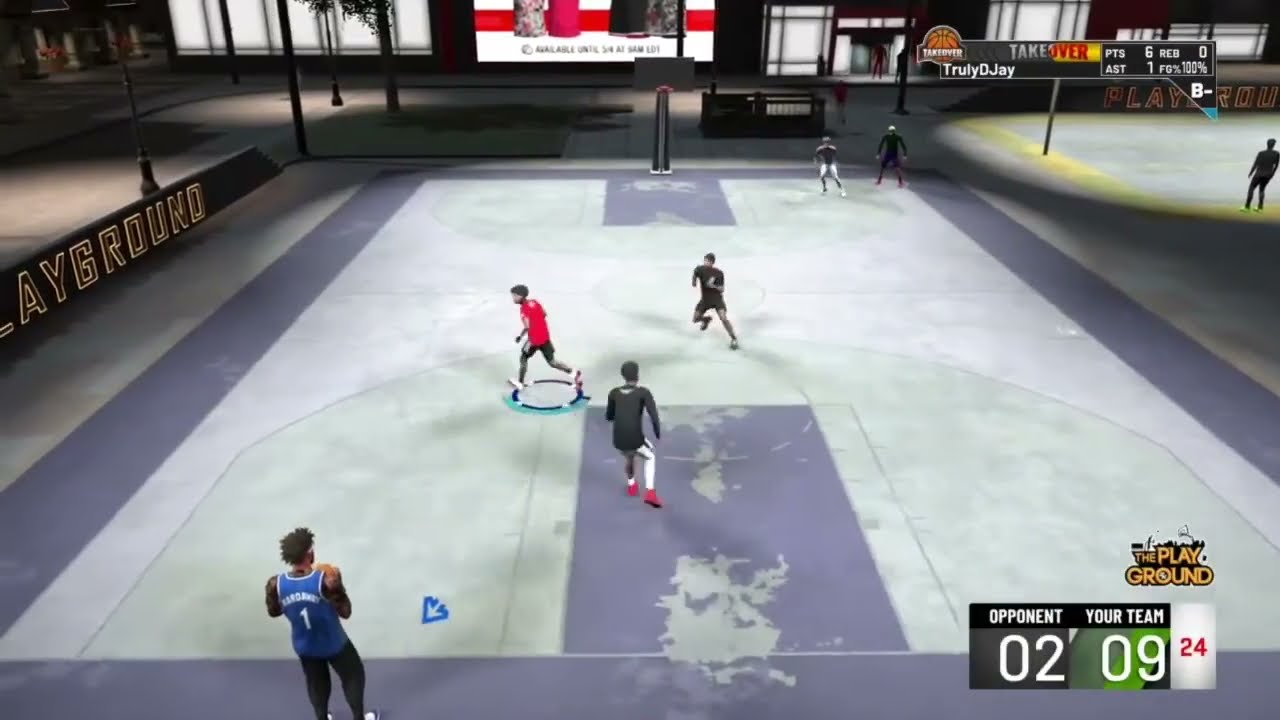This image is a detailed screenshot from a basketball video game set in an indoor court known as "The Playground." In the bottom right corner, the scoreboard shows "Opponent" with a score of 02 and "Your Team" leading with 09. A shot clock, highlighted in red, counts down from 24 seconds. Above the scoreboard, "The Playground" is prominently displayed in orange. The upper right section of the image features a player named "Truly DJ" with stats: 6 points, 1 assist, and a field goal percentage, along with rebound details.

The central basketball court is mainly gray with blue trimmings, worn down in areas to a lighter green and a purple-gray hue. Black light posts with shining lights illuminate the area. A player in the lower left corner wears a blue jersey with the number 1 and black pants. Nearby, other players include one in a red shirt and two in black jerseys. Additional players are visible in the distance on an adjacent court.

The background shows a detailed urban setting, including grass, subway station steps, buildings with lit entrances, and a billboard, adding to the immersive atmosphere of the game.